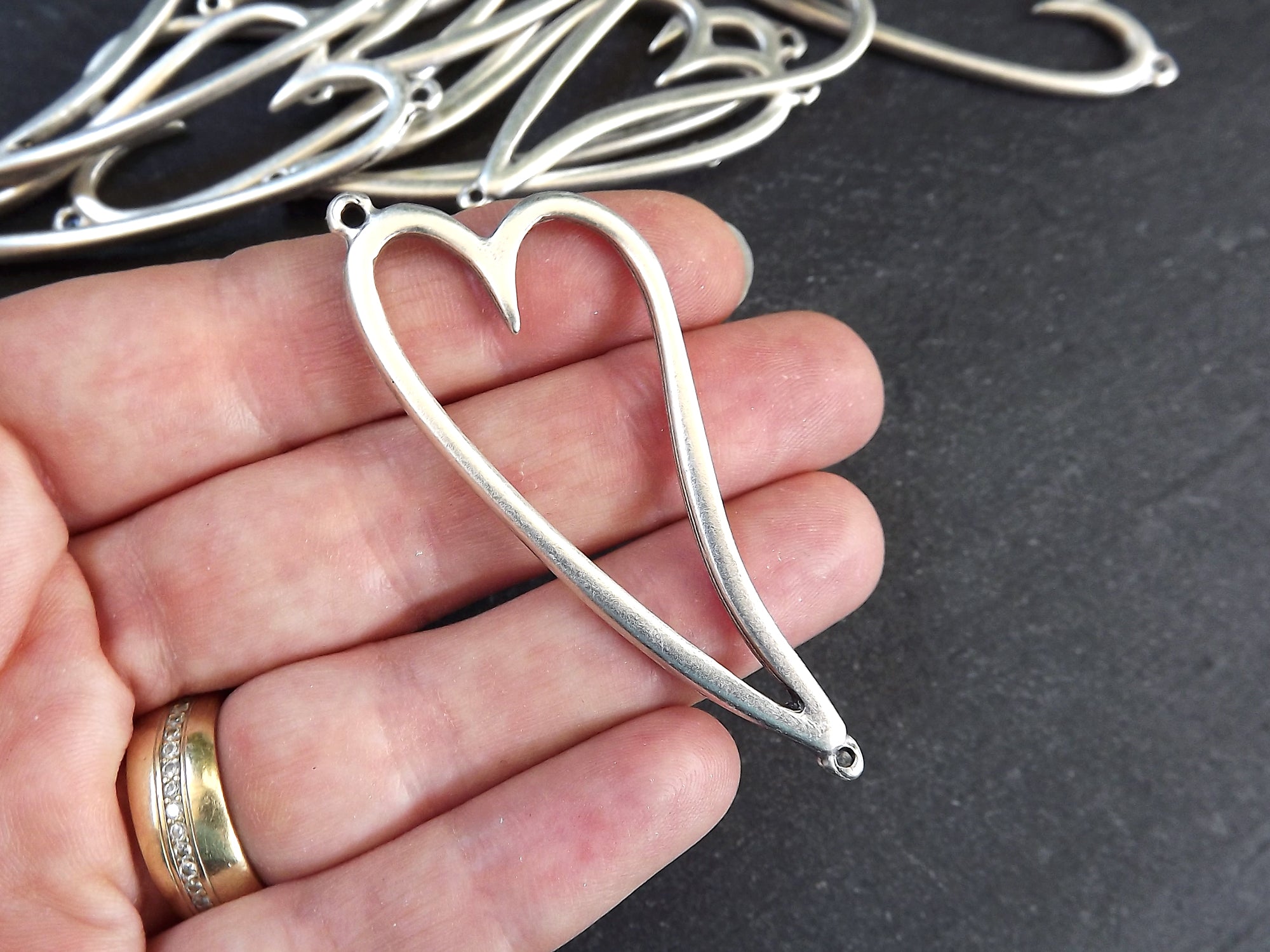In this close-up image, the palm side of a person's hand is visible, prominently displaying four white fingers while the thumb is out of view. Draped across the fingers, there's a silver heart pendant with an elongated, slightly curved, and slanted shape. The pendant features a round hole at the top, likely for attaching to a necklace or earring. The person is wearing a large gold band with a diamond center on their ring finger, and their hand rests on a black table. In the upper corner of the photograph, a pile of similar heart pendants can be seen. The fingertips, particularly the index finger, show a hint of fingernail. The detailed setting and positioning suggest the person, possibly selling these pendants, took the photo themselves.